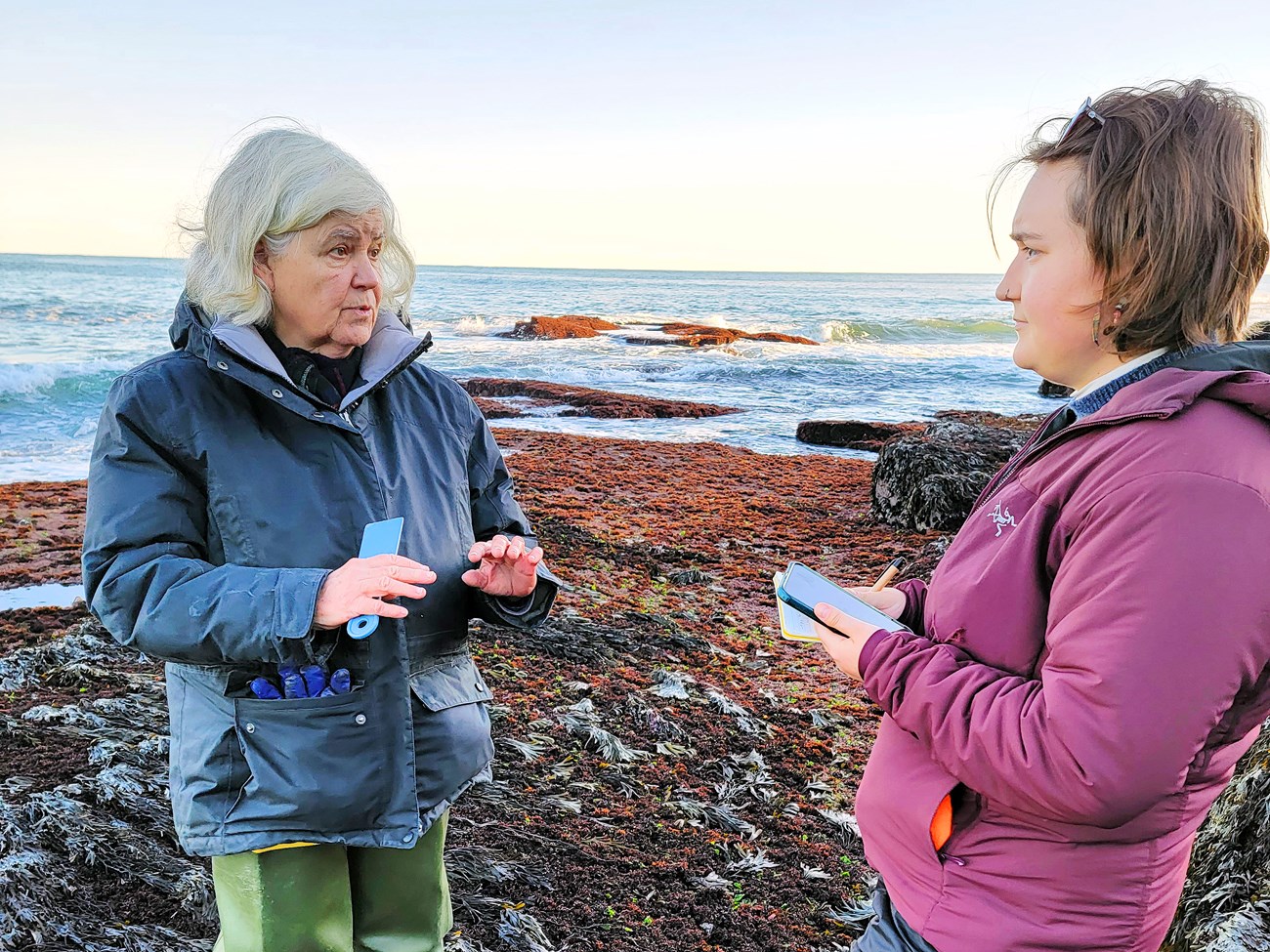In this photograph, two women are engaged in what appears to be an interview on a rocky, seaweed-covered section of a beach. The ocean is visible in the background with waves crashing over exposed rocks. The woman on the left is older, with shoulder-length white hair, and is dressed warmly in a dark blue, heavy jacket zipped up to her neck, with two large pouchy pockets from which the fingers of a bright blue glove are visible. She is holding a light blue scraper implement in her right hand and gesturing with her fingers outstretched, palms down. She is wearing green pants. The younger woman on the right has straight, short brown hair, and a nose ring, with glasses perched on top of her head, and an earring visible in her ear. She is also dressed warmly in a purple winter coat over a dark blue sweater and a white turtleneck. An orange object protrudes from her unzipped left pocket. She is holding a phone in her left hand and a notebook with a pen sticking up between her fingers in her right hand. Both women are focused on their conversation, with the older woman appearing to explain something while the younger woman listens intently. The setting could be a chilly, scenic coastal location such as Canada or Nantucket.